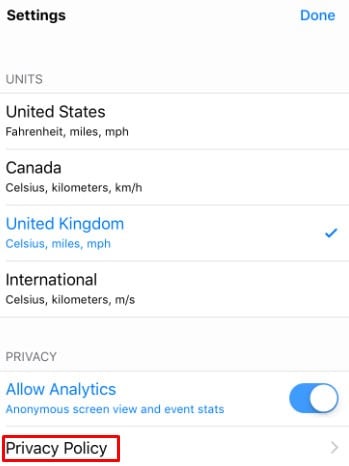### Detailed Caption:

This digital image displays a settings and privacy interface for a mobile application. At the top of the screen, the word "Settings" is prominently displayed in bold black font. To the right of this heading, there is a "Done" button shaded in blue. Below the heading, various units of measurement options are listed, categorized by regions:

1. **United States**: Listed with the following units - Fahrenheit for temperature, miles for distance, and MPH for speed.
2. **Canada**: Displaying units as Celsius for temperature, kilometers for distance, and KMH for speed.
3. **United Kingdom**: Marked with a blue checkmark indicating selection, showing units as Celsius for temperature, miles for distance, and MPH for speed.
4. **International**: Offering units as Celsius for temperature, kilometers for distance, and M/S for speed.

The section titled "Privacy" follows the units of measurement options. Under this section:

- **Allow Analytics**: This option is described as encompassing anonymous screen view and event statistics tracking and is currently selected, indicated by a blue highlight.
- **Privacy Policy**: This is noted in black font with an accompanying red check mark.

The options and settings appear organized within a rectangular boundary.